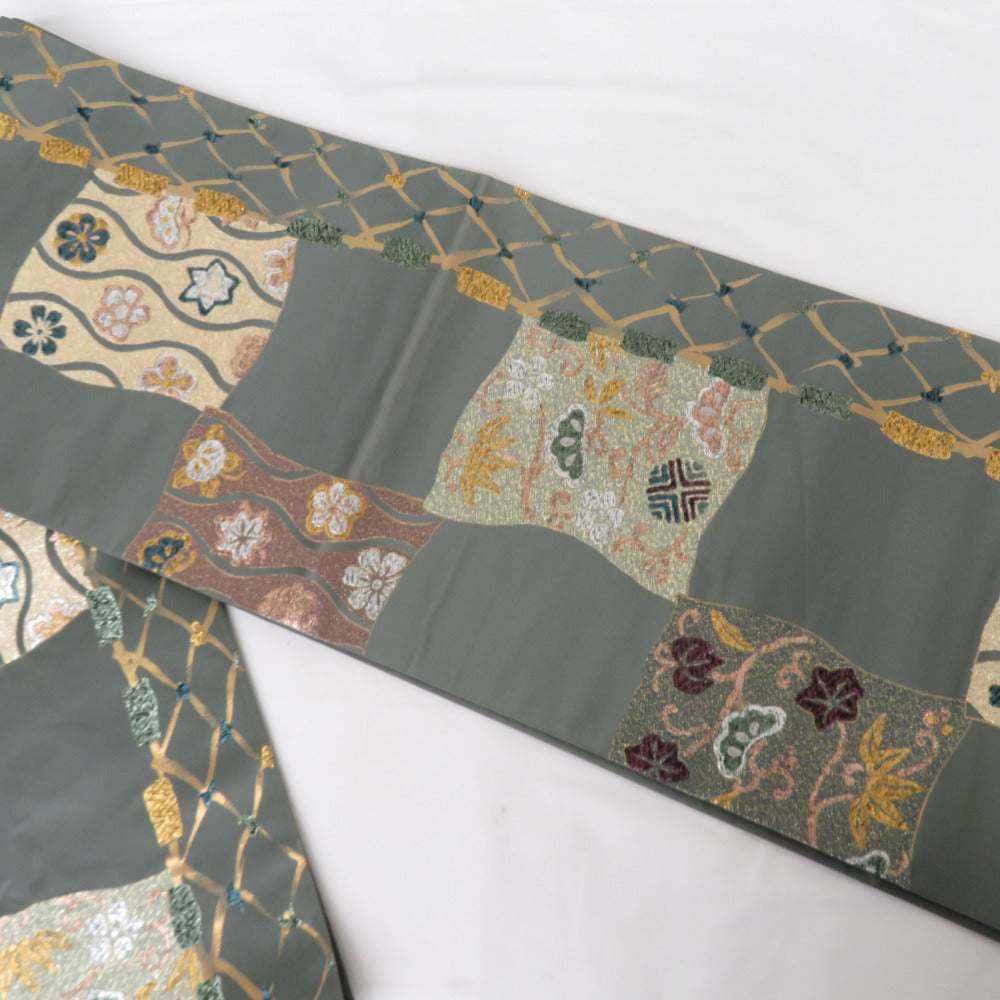This photograph features a detailed, handmade quilt laid out horizontally, showcasing intricate stitchwork and patchwork on a predominantly gray cloth. The quilt has a grayish-teal hue, with alternating sections of different floral designs in vibrant colors including red, white, pink, and gold, each set against unique colored backgrounds. The main body of the quilt is arranged in a checkerboard pattern, intermingling solid gray blocks with elaborately designed floral and leaf patterns, creating a visually rich tapestry. Along the side, there is a distinctive golden chain-link design offset to one edge, which adds an elegant touch. The quilt also has a border with a crisscross pattern, accented by small pops of yellow and light green, enhancing the overall decorative appeal. In the corner of the image, a second sheet of similar material is barely visible, suggesting an additional layer or companion piece to the displayed quilt.